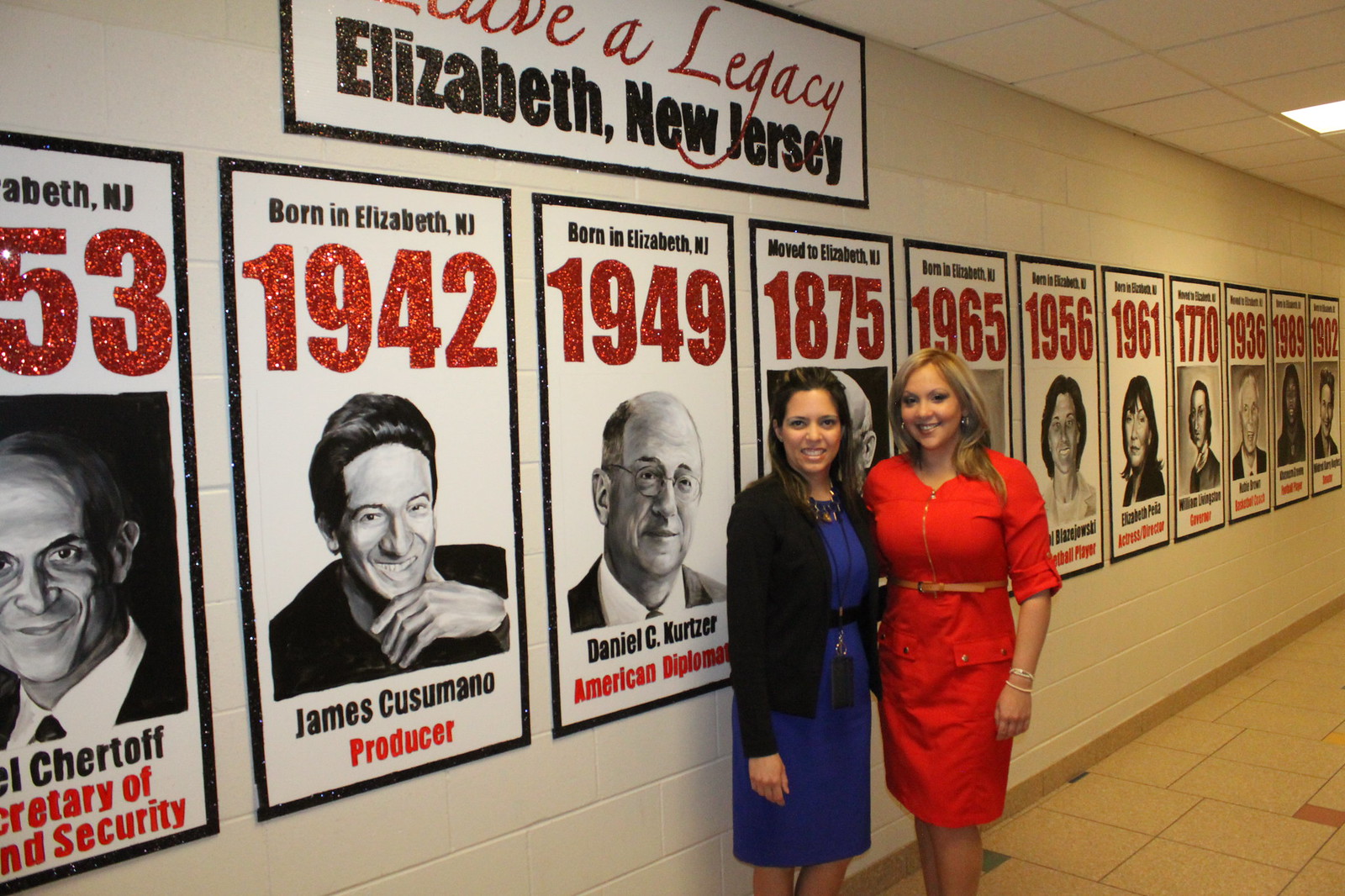In this horizontally aligned rectangular image taken inside a building with large white brick walls and light tan colored tile flooring interspersed with smaller colored sections, two women stand smiling in front of a commemorative wall. The wall, adorned with numerous vertical rectangular signs outlined in black, is crowned by the phrase "Leave a Legacy, Elizabeth, New Jersey." Each sign proudly displays glittery red years at the top, featuring notable individuals born in Elizabeth, New Jersey, along with their occupations. Prominent among these are signs for 1942 with a picture of James Cusimano, labeled as a producer, and 1949 with a picture of Daniel C. Kurtzer, identified as an American diplomat. The woman on the left, with long brown hair pulled back at the top, wears a blue dress paired with a black cardigan. Her companion on the right, with long blonde hair, is dressed in a red dress cinched with a tan belt. The wall extends further, showcasing additional people and their legacy from years ranging from 1875 to 1965. It’s likely the setting is a school, community center, or similar institution celebrating local history.